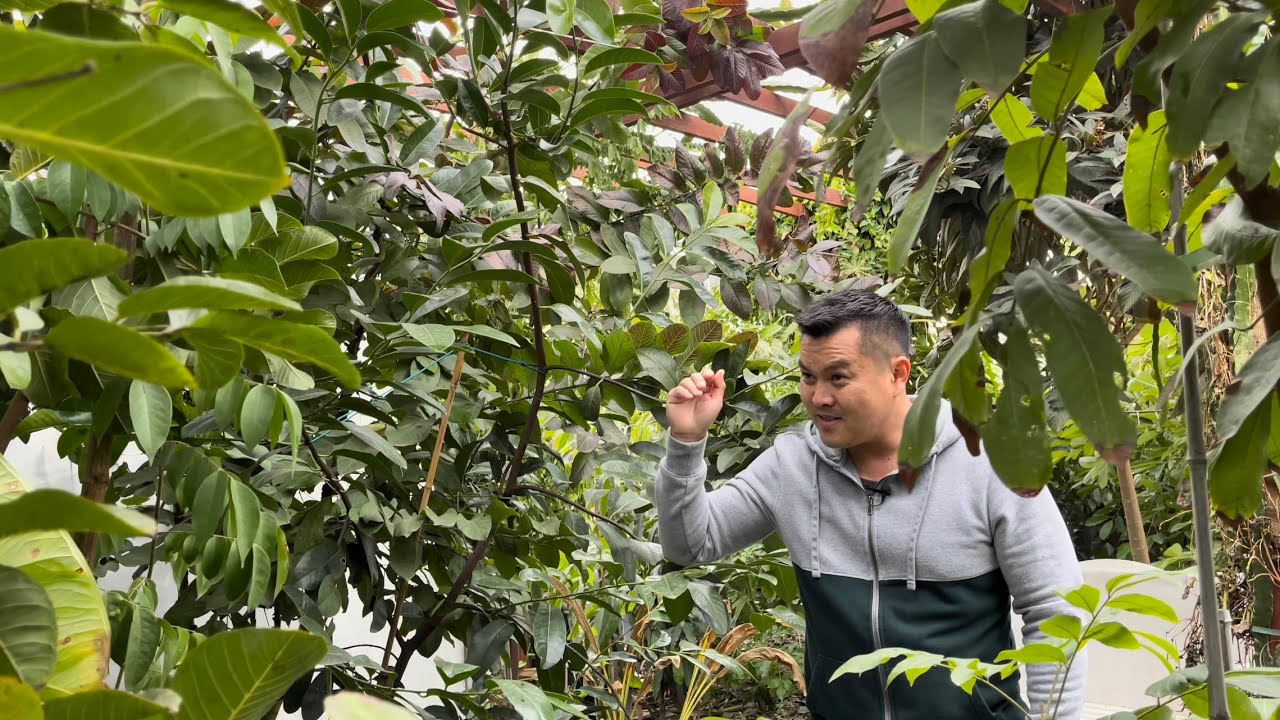The vibrant color photograph captures an Asian man in his 30s or 40s with a clean-cut hair that’s styled in a fade—short on the sides and longer on top. He is wearing a hoodie with a gray and black color scheme and a touch of forest green. The man stands just right of the center amidst a dense, plant-filled area that resembles a forest or a garden. He appears to be walking through, or perhaps pausing, to carefully examine a shrub with black branches and green leaves to his left. His right hand is held up, bent at the elbow, as he inspects a leaf with a thoughtful, perhaps concerned, expression on his face. Surrounding him are various trees and plants with tall stems and numerous branches laden with leaves. Above him, the sky is visible through what appears to be a wooden trellis, suggesting that the area might be part of a greenhouse or nursery rather than a natural forest. There's also a gray pathway visible in the background, adding to the structured setting amidst the lush greenery.